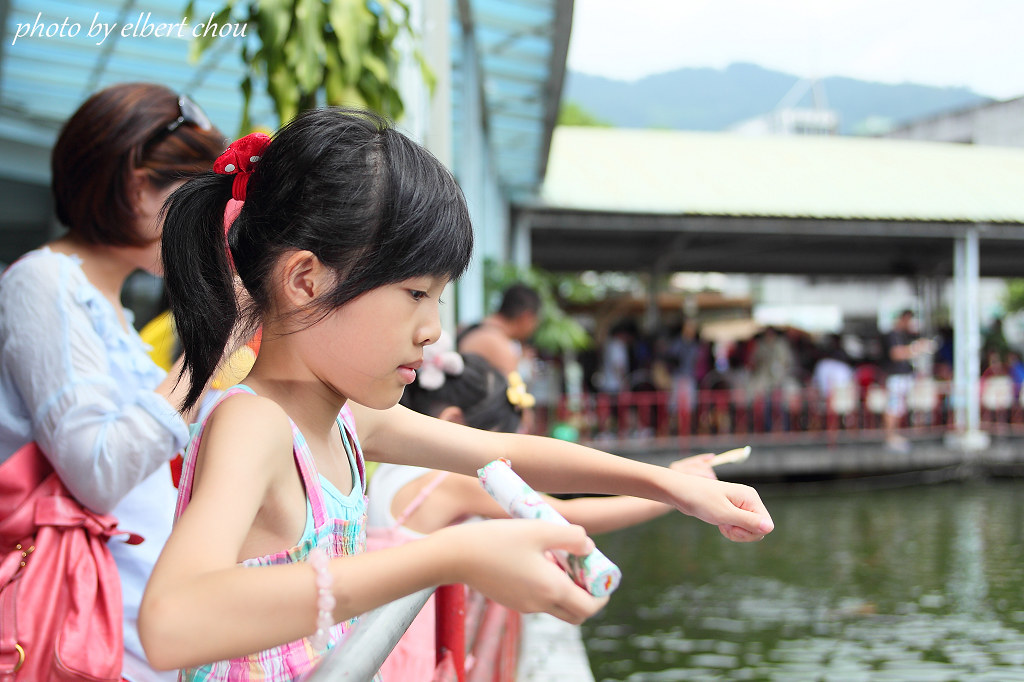This photograph captures a scene centered around a young Asian girl, around six or seven years old, who is the primary focus. The girl is standing in the foreground by a railing that overlooks a green body of water, possibly an aquarium. She has dark, nearly black hair pulled back into a ponytail with a red ribbon. She is clad in a pastel-colored blouse featuring shades of white, blue, and pink, and has straps over her shoulders. On her right wrist, she wears a bracelet and holds a cylindrical object with green and pink accents in her right hand, while her left hand is extended outward as if she is throwing something into the water. 

Behind her stands a woman, likely her mother, dressed in a white blouse and shouldering a blue handbag. Beside and beyond them, various blurred figures lean against the same railing, indicating a crowded setting. Above the young girl's head, green foliage hangs down, contributing to a natural ambiance. To the right, more blurred people can be seen lined up horizontally, accentuating the busy environment. The sky in the upper right corner appears bright blue with clouds, while the upper left corner shows a blue ceiling or umbrella. The image credit, "photo by Albert Chow," is indicated in white print in the upper left corner.